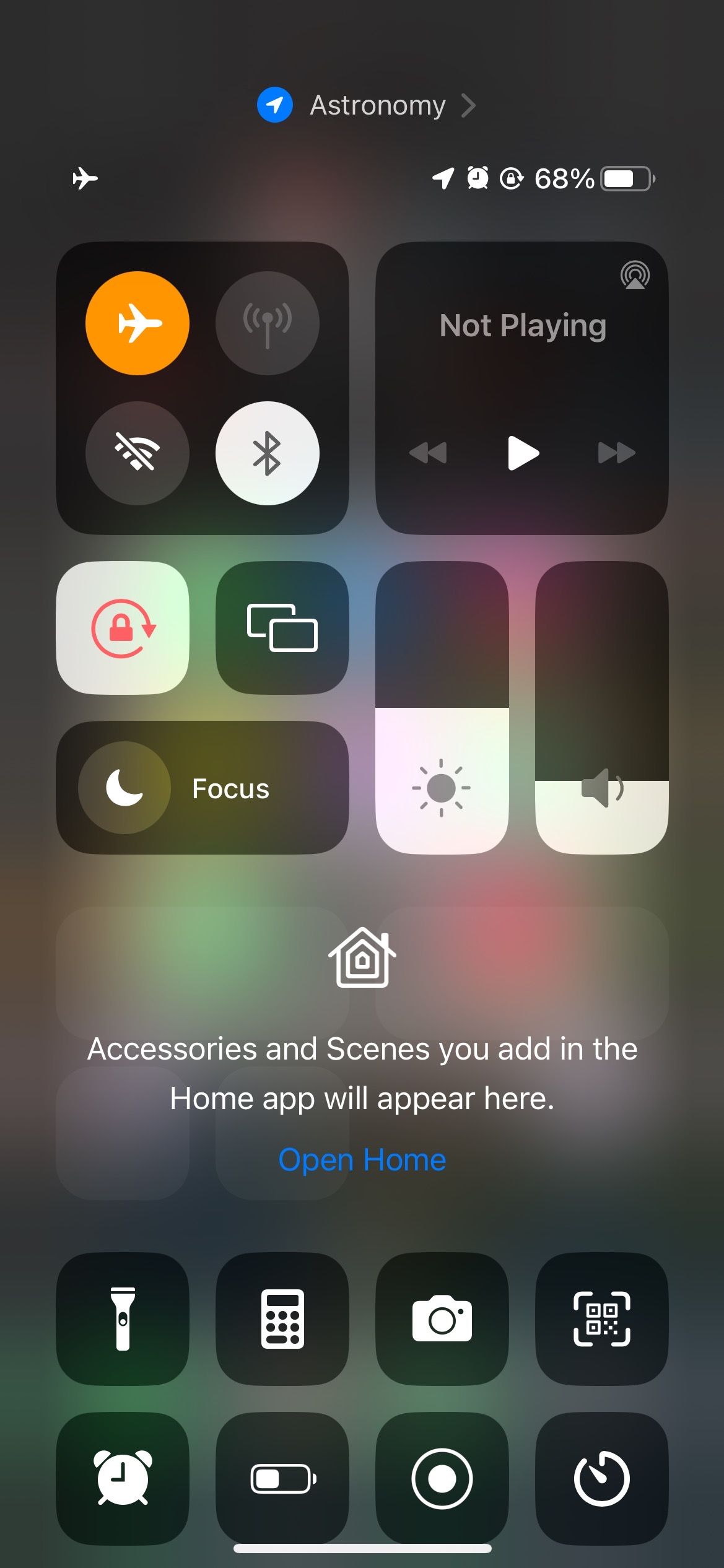In this image, the central focus is the word "Astronomy" prominently displayed at the top middle. To the left of the text, there's a blue circular icon with a white arrow pointing towards the top right. Adjacent to the word "Astronomy" on the right is a right-facing arrow. Below this, towards the right side of the image, there are several small icons in a row: a white arrow pointing to the top right, a clock icon, a lock icon, the battery percentage "68%", and a battery icon.

Beneath this row of icons, there are two distinct boxes. The left box features an airplane icon, a scratched-out Wi-Fi icon, a Bluetooth icon, and a phone signal icon. The box on the right displays the text "Not Playing," and below it, there are playback control icons: a play icon in the center flanked by two arrows on each side pointing outwards.

Further down the image, there are a few more boxes. In the middle right-side box, a volume icon indicates that the volume is set at about 20%. To its immediate left, a sun icon shows brightness set at approximately 40%. At the bottom of the image, the phrase "Open Home" is followed by the message "Accessories and scenes you add in the home app will appear here," accompanied by a small house icon.